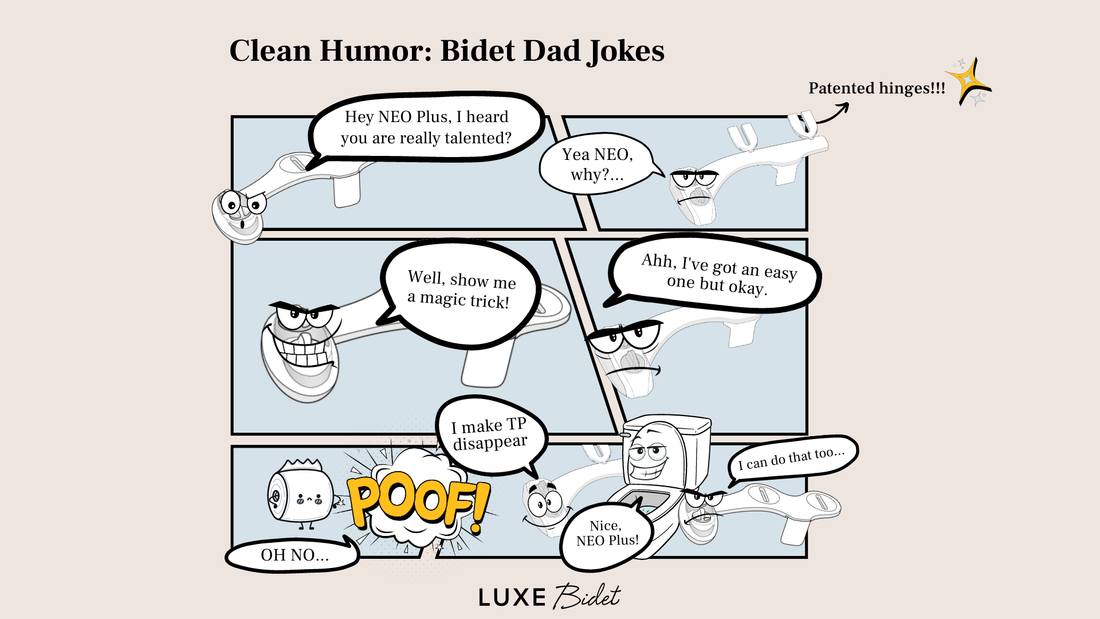This image is a comic strip style joke set against a beige background, titled "Clean Humor: Bidet Dad Jokes." The comic features various bathroom-related characters, namely two bidets, a toilet, and a personified roll of toilet paper, all illustrated in a muted color palette with some bright accents.

In the upper left panel, the Neo Plus bidet greets by saying, "Hey Neo, I heard you were really talented." The Neo bidet responds in the adjacent panel, "Yeah, Neo Plus, why?" In the middle left panel, Neo Plus, grinning, continues, "Well, show me a magic trick." Neo replies in the middle right panel with a slight smirk, "I've got an easy one, but okay."

The humor unfolds in the bottom left panel where a roll of toilet paper, illustrated with legs and a face, exclaims "Oh no!" as it is enveloped in a "poof," depicted by bright orangey-gold letters. In the final bottom right panel, the Neo bidet boasts, "I make TP disappear!" The toilet attached to Neo Plus compliments, "Nice Neo Plus," while the other bidet adds, "I can do that too."

At the bottom of the image, the branding "Lux Bidet" is prominently displayed, tying the humorous comic to the product being advertised.